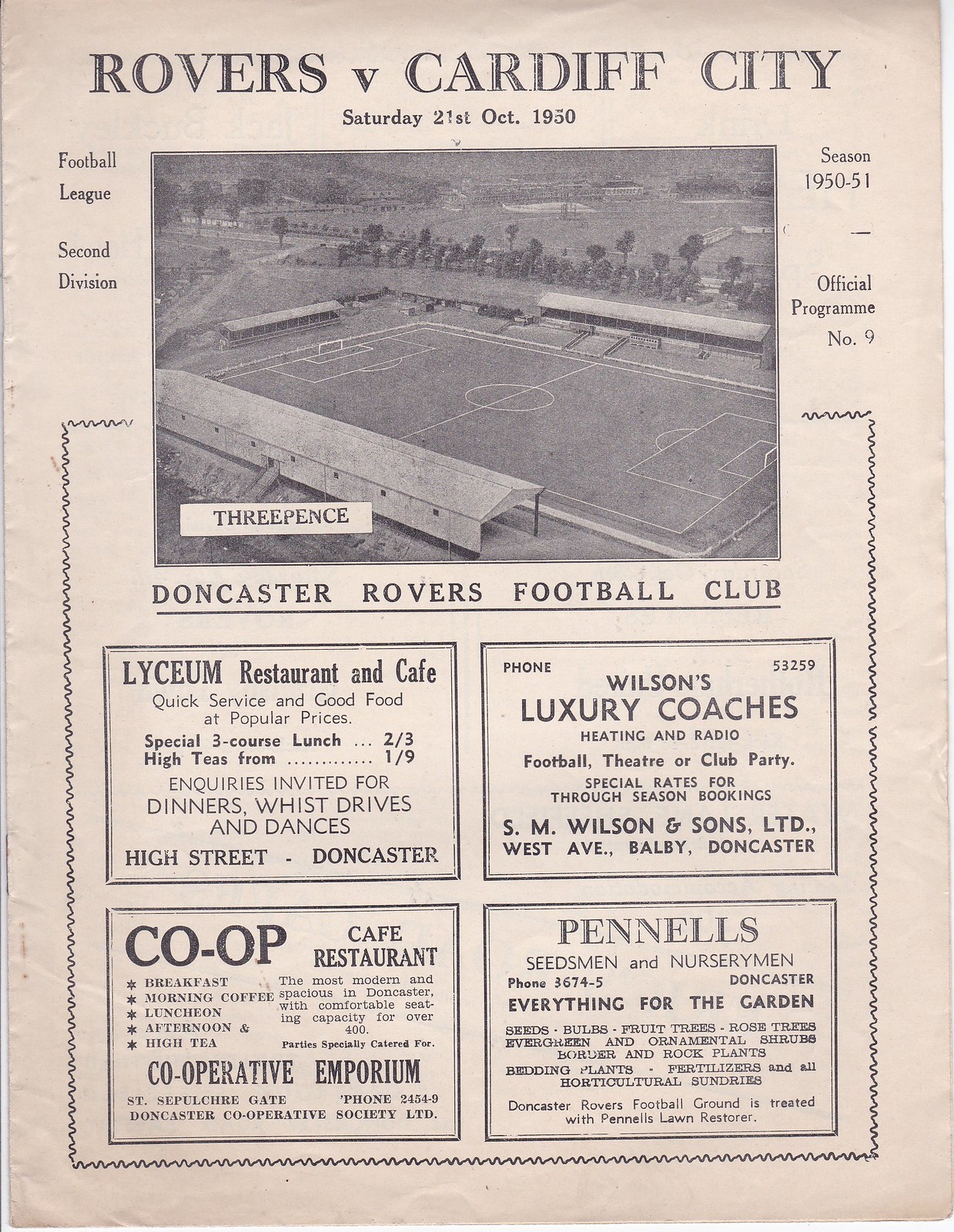This is a black-and-white soccer program cover for the match between Doncaster Rovers and Cardiff City on Saturday, 21st October 1950. The top of the page prominently features the title "Rovers vs. Cardiff City." Directly below, it mentions "Football League, Second Division, Season 1950-51 Official Program Number 9," and the cost is listed as three pence. The center of the page displays a faded, black-and-white photograph of a soccer field, with seating on three sides, trees behind the stands, and houses visible in the background. Below the image, the text reads "Doncaster Rovers Football Club" in bold lettering. Further down are four rectangular advertisements: the upper left advertises the Lyceum Restaurant and Cafe for quick service and good food at popular prices; the upper right features Wilson's Luxury Coaches, highlighting heating, radio, and special rates for seasonal bookings; the lower left promotes the Co-op Cafe Restaurant offering various meals and teas; and the lower right showcases Pennell's Seedsmen and Nurserymen, providing everything for the garden.